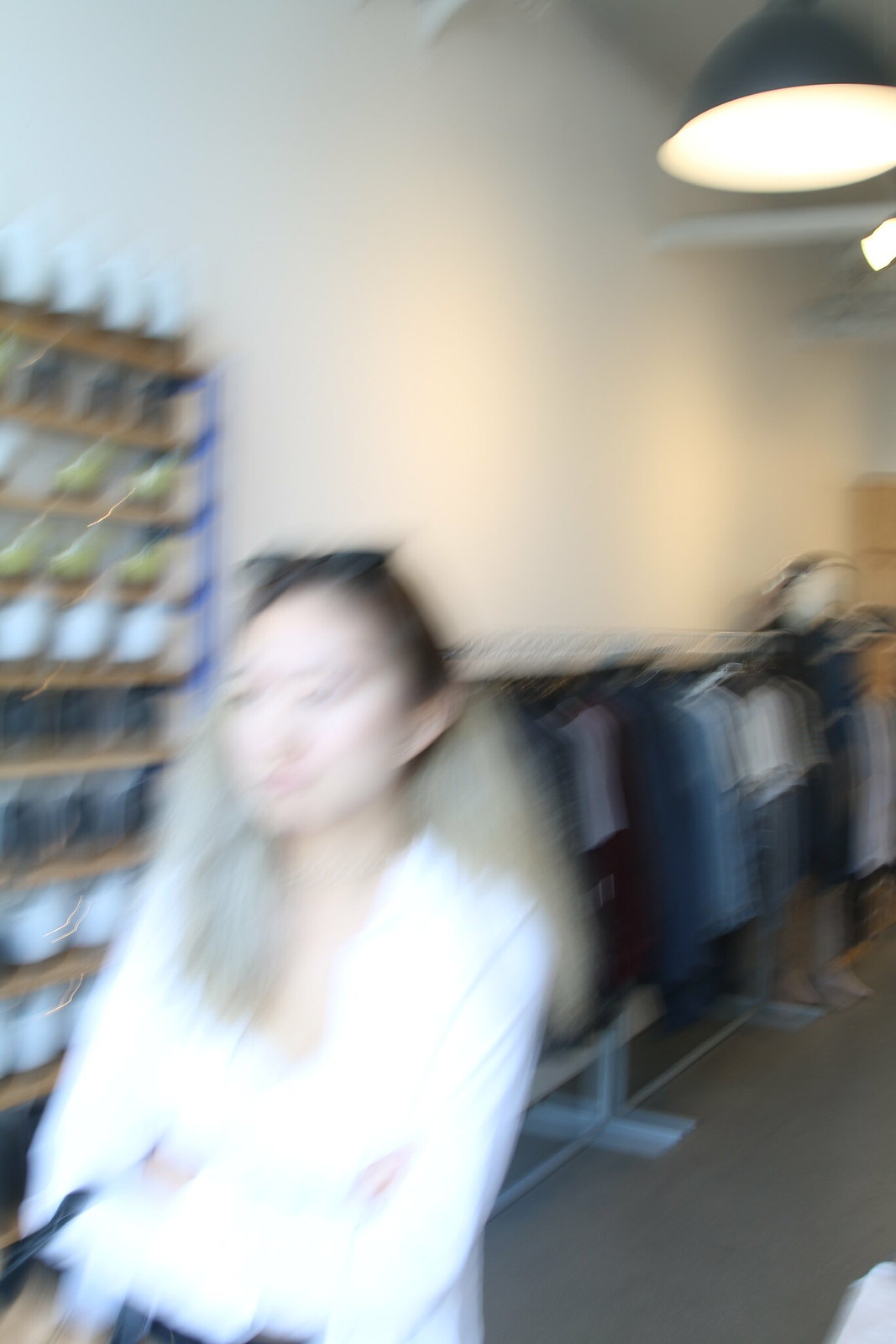This blurry photograph captures the interior of what appears to be either a store or an individual's closet. The image seems to have been taken in motion, likely causing its lack of clarity. On the left side of the picture, there is a woman with long blonde hair. She is dressed in a long-sleeved white shirt and either dark pants or a skirt. To her left is a shelving unit stocked with various pairs of high-heeled shoes in colors ranging from white to gray to gold. Additionally, behind the woman, there is a row of clothing hanging on a long rack. The room itself is painted white and features a dark gray carpet.